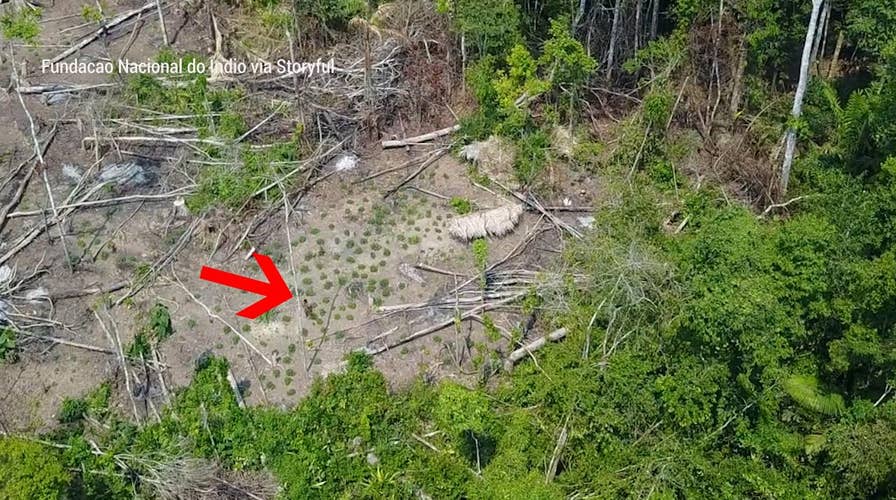This aerial photograph showcases a forested area, encircling a large, barren clearing marked by numerous fallen and dead trees, starkly contrasting with the dense green vegetation surrounding it. The scene, likely captured by a map service like Apple Maps or Google Maps, hints at a possible natural disturbance, such as a flood, that has left the central area stripped of vegetation, littered with gray sticks and thin logs. Prominently featured in the left third of the image is a red arrow, directing attention to small round clusters of green amidst the desolation. Above this arrow, text in Spanish or Portuguese reads "Fundação Nacional do Índio via Estorvo," suggesting the source of the image. The photograph poignantly highlights the boundary between the verdant forest and the impacted clearing, emphasizing the stark difference in vegetation density.